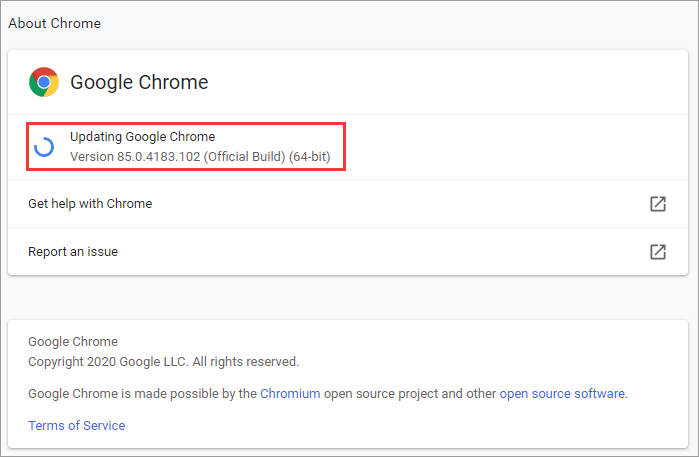The image displays the Google Chrome update page, prominently featuring the familiar multi-colored red, blue, yellow, and green circular logo at the top. It indicates that the browser is currently being updated to version 85.0.4183.012. Beneath this update status, two actionable links are provided: 'Get help with Chrome' and 'Report an issue,' guiding users to additional support options as needed. At the bottom of the screen, the page notes Google Chrome's copyright details, stating, "© 2020, Google LLC, all rights reserved." It acknowledges that Google Chrome is made possible by the Chromium open-source project, along with other open-source software contributions. The footer also includes a clickable blue 'Terms of Service' phrase for those interested in the legal aspects of the software. Overall, the image suggests that users should prepare for a brief wait as the update process completes.